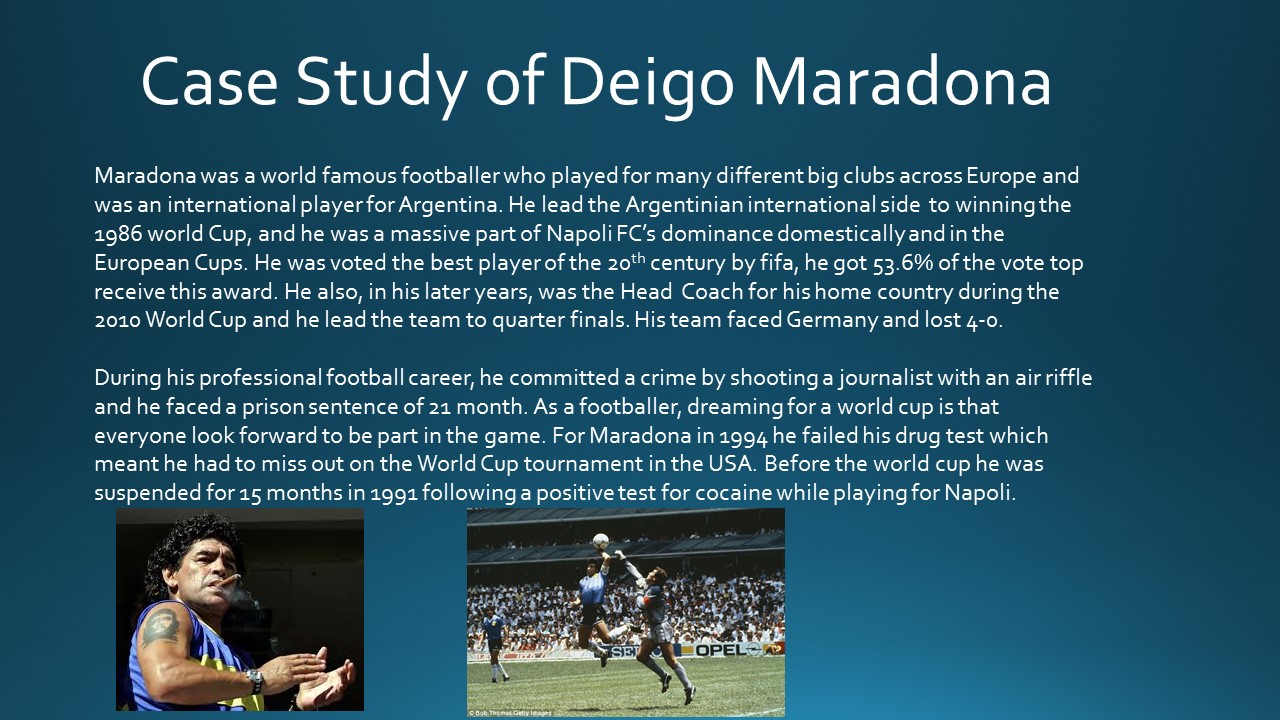The image features a half-page magazine layout with a dark blue background and white text, prominently titled "Case Study of Diego Maradona." Two color photographs adorn the lower section of the page. On the left, there is an image of Maradona, sporting a blue sleeveless shirt that reveals a Che Guevara tattoo on his shoulder. He is captured smoking a cigar and appears to be clapping, his gaze directed downward. The second photograph, positioned in the center, depicts Maradona in action during a soccer match, leaping to head the ball, with a packed stadium full of spectators in the backdrop.

The accompanying text provides a detailed account of Maradona’s illustrious career and personal controversies. It emphasizes his global fame as a football player who led Argentina to victory in the 1986 World Cup and significantly contributed to Napoli FC's success in Europe. Notably, Maradona was voted FIFA's best player of the 20th century with 53.6% of the vote. However, his career was also marred by legal issues, including a 21-month prison sentence for shooting a journalist with an air rifle, and multiple drug-related suspensions, including a 15-month ban in 1991 for a positive cocaine test while playing for Napoli, and being banned from the 1994 World Cup following another failed drug test.

Despite the acclaim and accolades, the text also reveals some typographical errors, such as the misspelling of Maradona's name as "Deigo." The overall design combines photographic representationalism with stylish typography, presenting a compelling and multifaceted portrait of the legendary footballer.